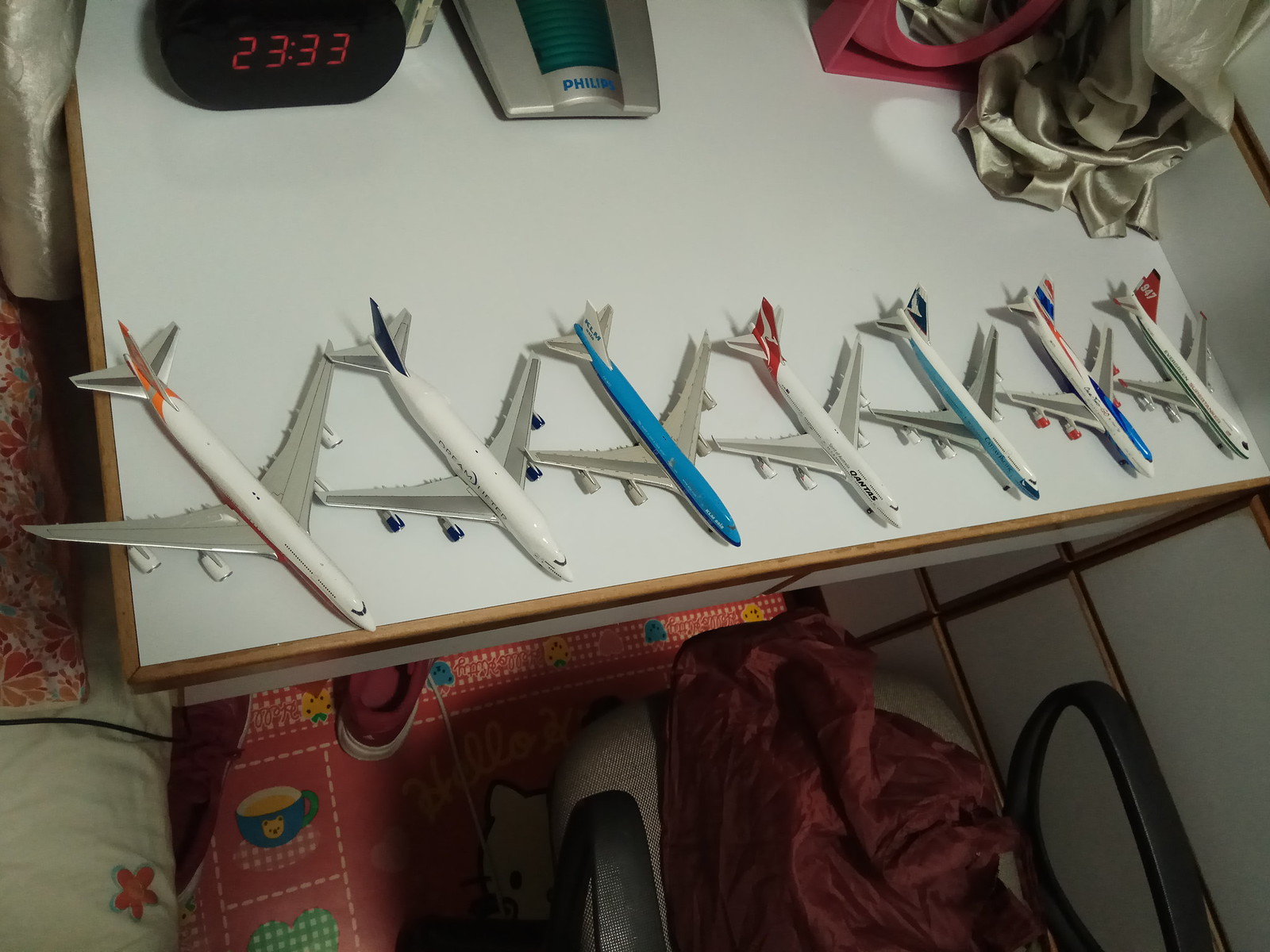The image depicts a white nightstand with a light wood trim, holding a collection of seven model airplanes meticulously lined up from largest to smallest. Each plane, made of plastic, features a distinct color scheme and branding details. Starting from the left, the planes present a range of colors including a white plane with an orange tail, a white plane with a black tail, a blue-bodied plane with a white tail, a white plane with a red and white striped tail, a white plane with an aqua blue stripe, a white plane with blue, red, and white stripes, and finally, a white plane with a red tail. The table also holds a Philips alarm clock that is silver with a green display, as well as a magnifying mirror with a pink frame. Below the nightstand, a pink patterned sheet covers what appears to be a bed, over which a silky blanket and a single pink shoe are casually placed. Adjacent to the nightstand, white bed sheets adorned with a pink star and a pink pillowcase are visible.